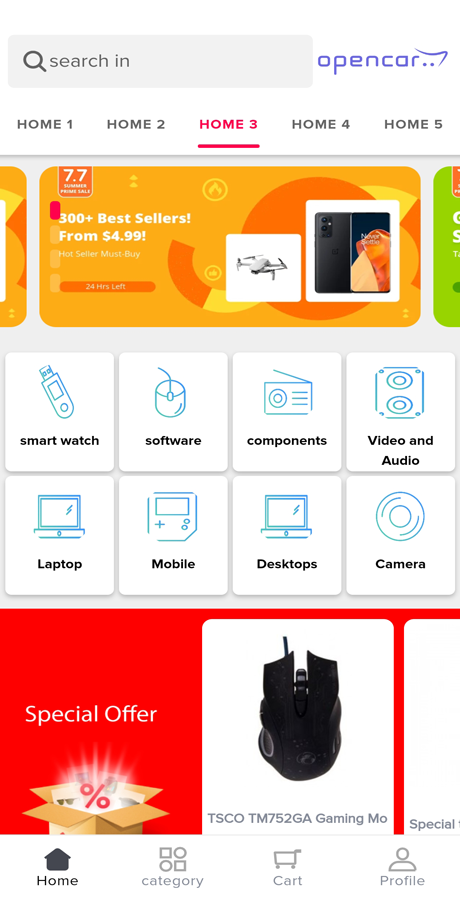The image depicts a smartphone screen showcasing a search page. The layout is predominantly on a white background. 

At the top, it says "Search in" followed by the phrase "Open Car." Below this, there are options labeled "Home 1," "Home 2," and "Home 3," with "Home 3" highlighted in red, while the others are in black. Following these are "Home 4" and "Home 5," also in black.

Further down, a place is rated 7.7 out of 10, alongside a mention of "300+ best sellers from $4.99." A prominent button is situated below this text. The button is housed within an orange box with subtle tinges of red.

Beneath the button, additional categories are listed: "Smartwatch," "Software," "Components," "Video and Audio," "Camera," "Desktops," "Mobile," and "Laptop." There's a "Special Offer" section prominently displayed in a red box. Within this red box, "Special Offer" is written in white text and accompanied by an image of a red percentage sign.

Encased within these elements are lines framing a TSCO gaming module. At the bottom, navigation icons for "Home," "Category," "Cart," and "Profile" are visible.